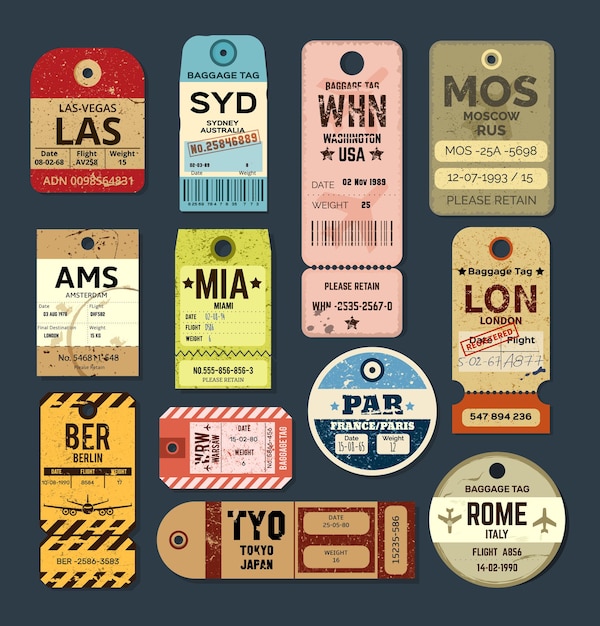The image showcases a collection of diverse luggage tags arranged against a dark blue backdrop. These tags, varying in color, size, and shape, represent destinations from around the globe. At the top left, a red and white tag from Las Vegas dated 1968 stands out. Next to it is a blue and white tag from Sydney, and a pink tag from Washington, USA dated November 2, 1989. Continuing to the right, there's a gray tag from Moscow dated December 7, 1993. In the second row, a brown and white Amsterdam tag leads, followed by a green Miami tag, both with unreadable dates, and a reddish Warsaw tag with the date 1528A. The third row features a yellow and black Berlin tag, a red and green horizontal tag from Tokyo marked 255A, and a light blue and dark blue Paris tag proclaiming 15165. The final row includes a silver tag from Rome dated February 14, 1990, while a cream London tag from May 2, 1967 sits to the left, and directly above these, a prominent yellow and black Berlin tag mirrors a warning sign. Each tag reveals signs of wear, evoking a sense of history and travel.